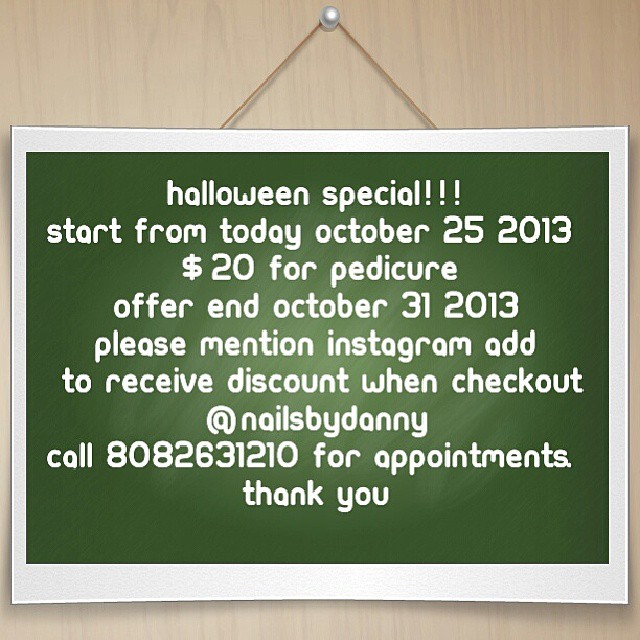This computer graphic advertisement features a green chalkboard-style sign with white text highlighted by a thin white border, giving a clean and classic look. The sign is suspended from a string held up by a thumbtack, positioned against a wooden background. Prominently, the sign displays "Halloween Special!!!" in all lowercase letters, announcing a discount offer from October 25th, 2013, to October 31st, 2013. The promotion is for a $20 pedicure at Nails by Danny, and customers are instructed to mention the Instagram ad at checkout to receive the discount. For appointments, the contact number 808-263-1210 is provided. The detailed and nostalgic design, dating back nearly a decade, adds a charming touch to this Halloween-themed special.